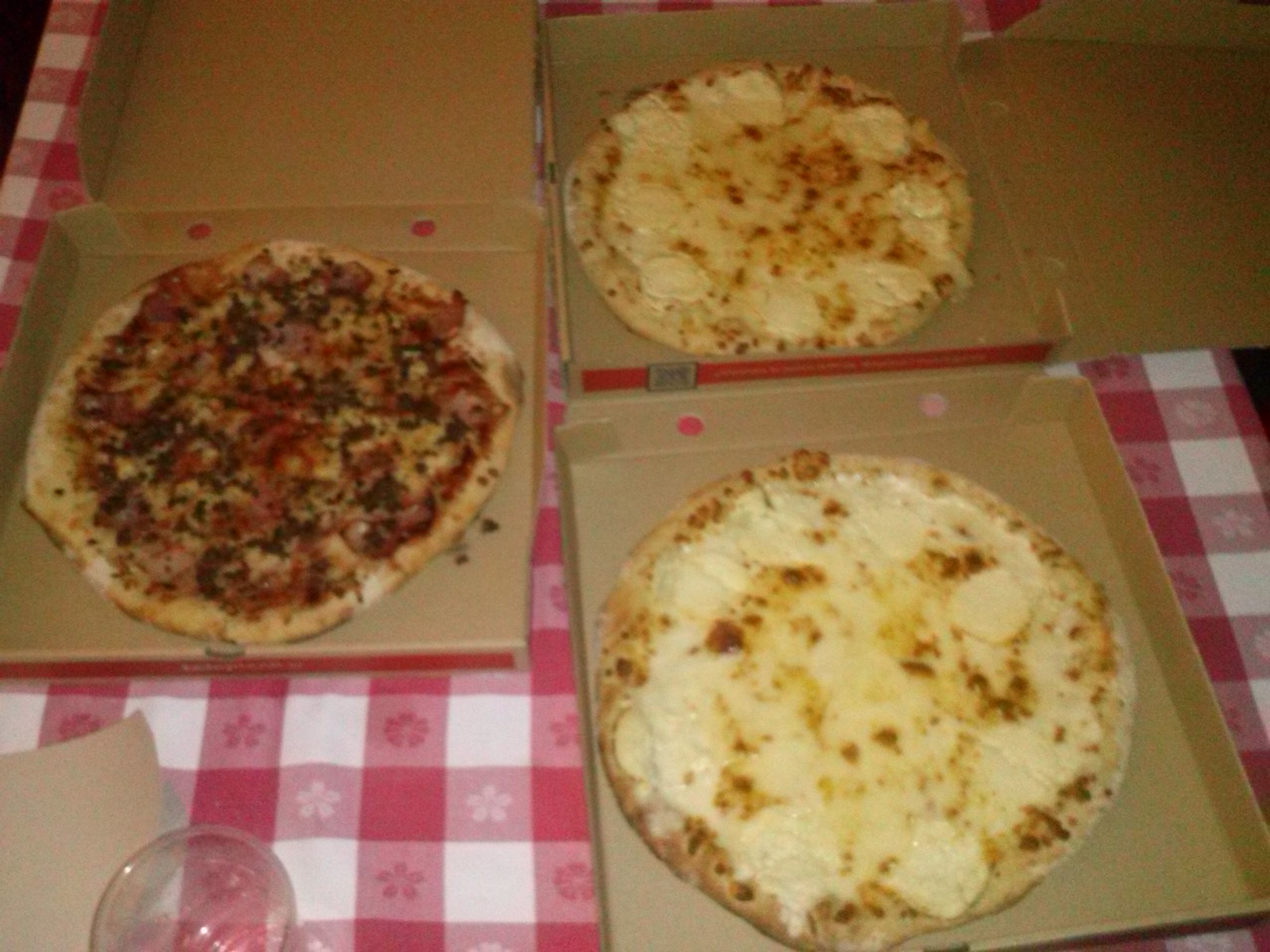This is a color photograph taken from a slightly angled top-down view, showcasing three open pizza boxes arranged on a red, white, and pink checkered tablecloth decorated with five-sided flowers in every other square. The pizzas are positioned to form a triangle, pointing towards the nine o’clock direction. The right side of the image displays two round cheese pizzas in cardboard boxes; one is in the lower right corner and another just above it, with the lid hanging off to the right. Both cheese pizzas appear to be whole and barely sliced, if at all. The pizza box on the left contains a combination pizza with a variety of toppings, including distinct colors of red, green, yellow, and brown, suggesting ingredients like pepperoni, sausage, black olives, and green peppers. Additionally, in the foreground of the lower left part of the photo, there is a brown napkin and a clear, empty glass.